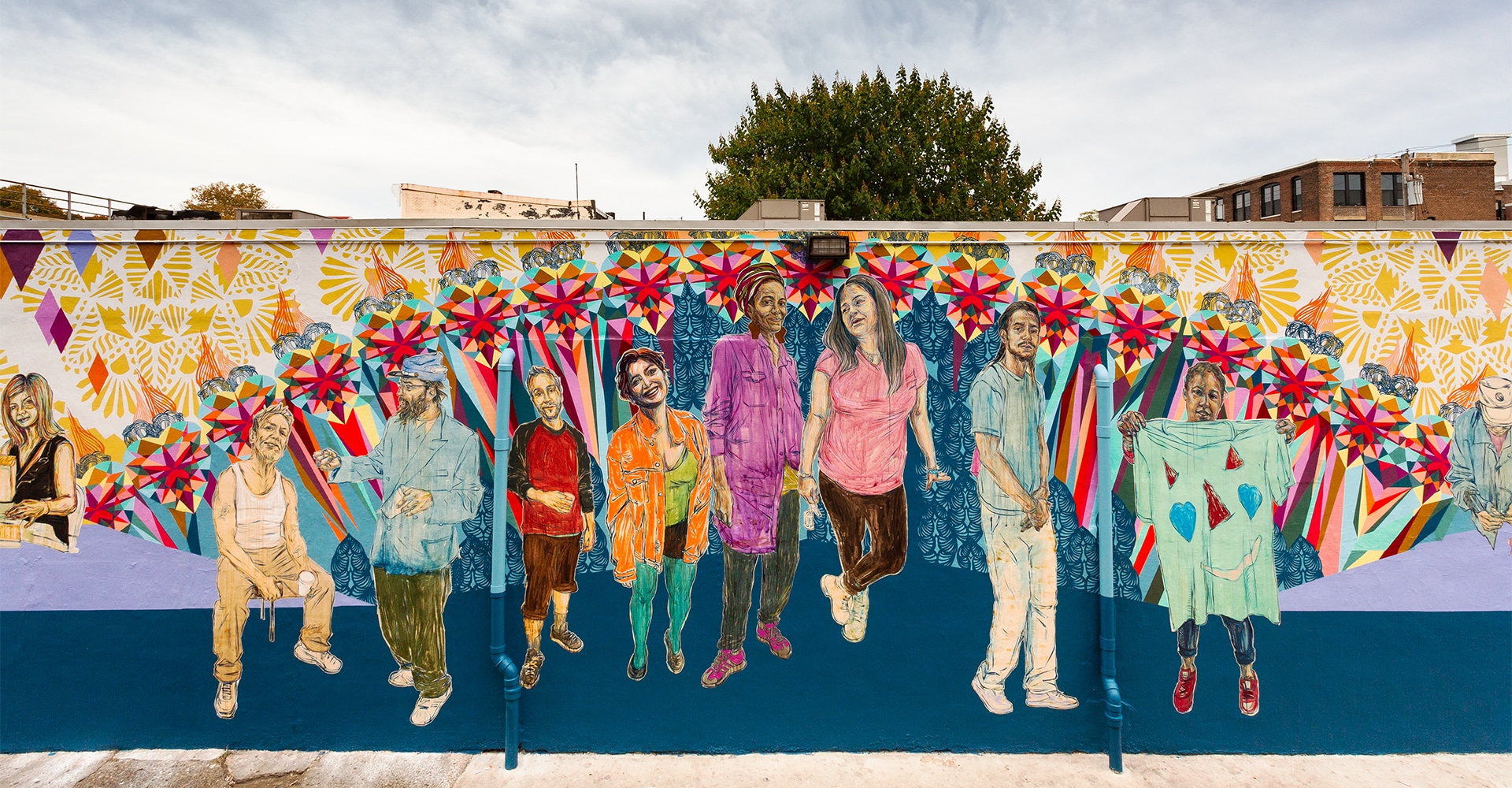This vibrant city mural, captured in a photograph, showcases an array of figures painted on an outdoor wall, possibly in a neighborhood setting. The mural features various people, primarily young, both standing and sitting, amidst an intricate background adorned with colorful patterns. On the far left, a young woman with long hair and a black shirt appears to be working at a computer terminal, surrounded by gold flowers. Next to her, a man in a white tank top, tan pants, and white tennis shoes sits on a bench. To his right stands a young male in a red and black baseball jersey and black pants that extend slightly below his knees.

Further along, another man is depicted in a blue baseball hat, a blue sport coat, green pants, and white shoes. The mural also includes an older male with a beard and glasses, several young females, and another figure on the far right who appears to be looking down at their hands. Above these figures stretches an arch adorned with stars in red, pink, and gold hues, accompanied by various shapes such as blue, purple, and red diamonds. The background is a dark blue surface with light blue elements, forming an almost surreal and richly detailed artistic scene.